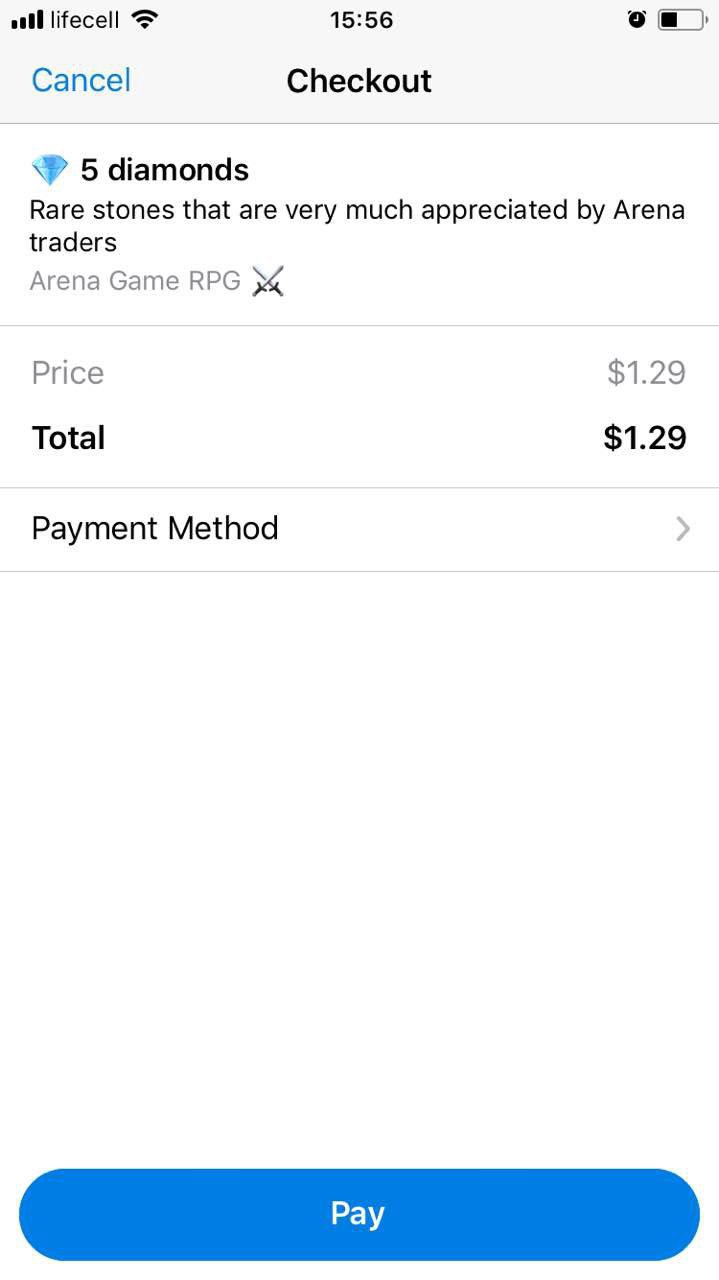The mobile screenshot captures a checkout page from an app, likely a game or an e-commerce platform. At the top of the screen, the status bar indicates the phone carrier is LifeCell with full signal strength (four out of four bars) and full Wi-Fi connectivity. The time shown is 3:56 PM, represented as 1556, and the battery level appears to be around 35%, indicated by an icon. 

In the upper center of the screenshot, the page title "Checkout" is prominently displayed. In the top left corner, a blue "Cancel" button allows users to exit the checkout process. Below this, a section features "5 Diamonds" alongside a sparkling blue crystal-cut diamond emoji. The text underneath reads, "Rare stones that are very much appreciated by arena traders." This is followed by the label "Arena Game RPG" with an icon of two crossed swords, symbolizing the game's genre.

The cost of the purchase is clearly listed as $1.29, with both the price and total displayed; the price is in gray and the total in black, providing clear differentiation. Below these details, the label "Payment Method" is in black, accompanied by a right-facing gray arrowhead suggesting a link to select or change the payment option.

A considerable amount of white space separates these details from the "Pay" button at the bottom of the screen. This button is capsule-shaped, blue, and features the word "Pay" in white font, making it stand out as the call-to-action for completing the transaction.